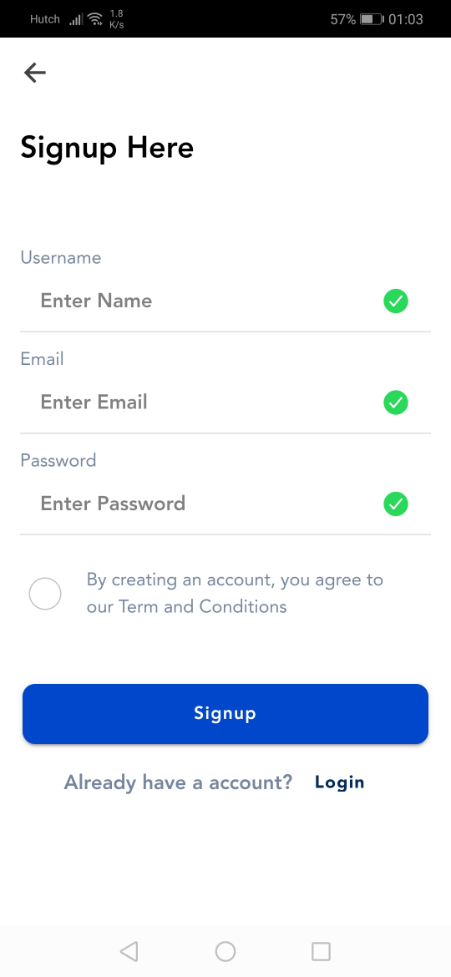A detailed screenshot of a mobile phone's sign-up interface, with key elements highlighted:

1. **Top Status Bar**:
   - **Background Color**: Black
   - **Text Color**: Gray
   - **Left Side**: Network provider name "Hutch", full-strength cell service icon, full-strength Wi-Fi icon, and a data transfer rate displayed as "1.8 K/S".
   - **Center**: Blank black space
   - **Right Side**: Battery icon displaying 57% charge. Time displayed as "01:03" in gray text, indicating 1:03 AM.

2. **Main Screen**:
   - **Background Color**: Predominantly white
   - **Text Color**: Black
   - **Navigation Arrow**: A black arrow pointing to the left at the top of the screen.

3. **Sign-Up Form**:
   - **Sign-Up Text**: "Sign up here" in black on the left.
   - **Username Field**: Label "username" in gray, with an empty white entry field beneath it showing "enter name" in gray.
   - **Verification**: A white checkmark on a green background located to the right of the username field.
   - **Email Field**: Similar format as the username, with the label "email" in gray and an entry field showing "enter email" in gray.
   - **Password Field**: Label "password" in gray, with the entry field showing "enter password" in gray.

4. **Terms and Conditions**:
   - **Text**: "By creating an account you agree to our terms and conditions," in gray text at the center, accompanied by a small circle icon to the left.

5. **Sign-Up Button**: 
   - **Design**: A blue rectangle containing the word "sign up" in white, centered within the button.

6. **Additional Options**:
   - **Support Phrase**: "Are we having a question?" in blue text beneath the sign-up button.
   - **Login Option**: "Login" in black text is located to the right of the support phrase.

7. **Footer Icons**:
   - **Icons**: A gray triangle pointing to the left, a circle, and a square, aligned horizontally and located at the bottom of the screen. 

This detailed caption encapsulates the visual and functional aspects of the mobile sign-up interface.